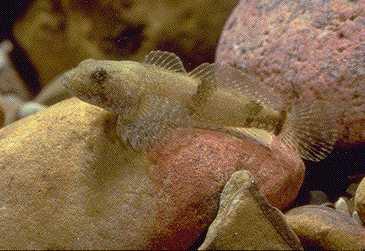This close-up image captures a uniquely shaped fish perched on a large, dual-colored rock within a rocky riverbed. The fish exhibits a remarkable camouflage, blending seamlessly with the pink and red hues of the rock it rests on. Its body is primarily yellowish and brownish with three distinct vertical stripes, and it has speckled black eyes. The fins and tail are translucent with thin white lines radiating outward, allowing the background to show through and adding to its harmonious appearance with the surroundings. The rock below the fish transitions from earthy brown-yellow on the left to vibrant pink and red on the right, while more medium-sized, smooth rocks and hints of additional colors like blue appear in the background, creating a vibrant, aquatic scene.